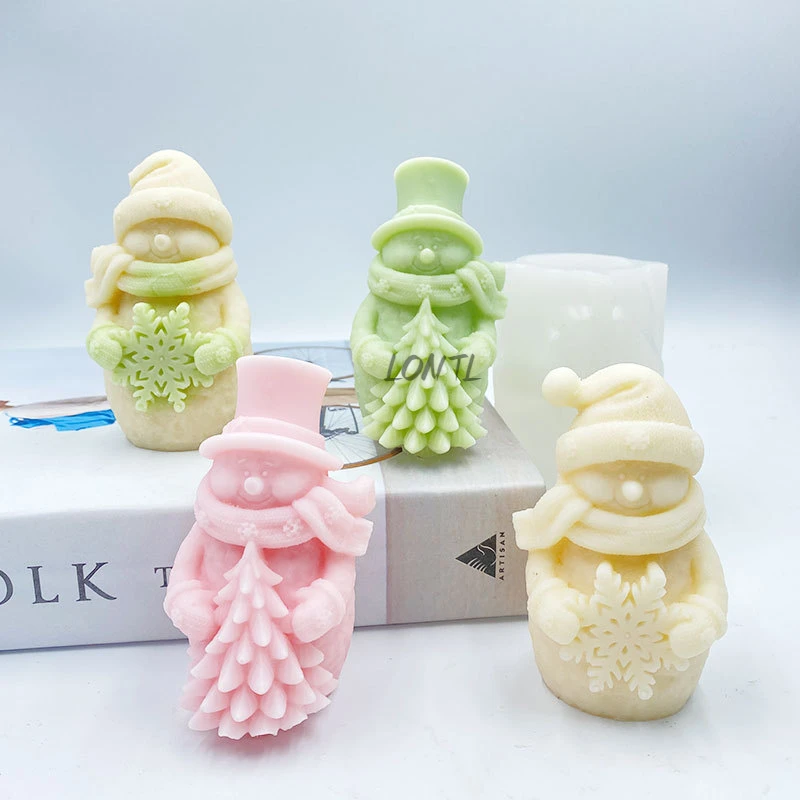This color photograph, presented in a square format, features four detailed wax soap figurines shaped like snowmen, each adorned with seasonal accessories. The snowmen are vibrant in color, including pink, white, green, and a peachy-orange hue. They are distinguished by their unique attire and the items they hold: two hold Christmas trees, while the other two clutch large snowflakes. The snowmen have different hat styles; two wear top hats, and the other two sport Santa Claus-style toboggan hats. Each snowman also dons a scarf wrapped around its neck. The snowmen are displayed atop a holder, which seems to advertise their purpose, with partial letters "O," "L," and "K" visible, possibly associated with the Artisan brand. A small candle can be seen nearby, and the entire setup is arranged on a white surface, giving the scene a festive holiday atmosphere.